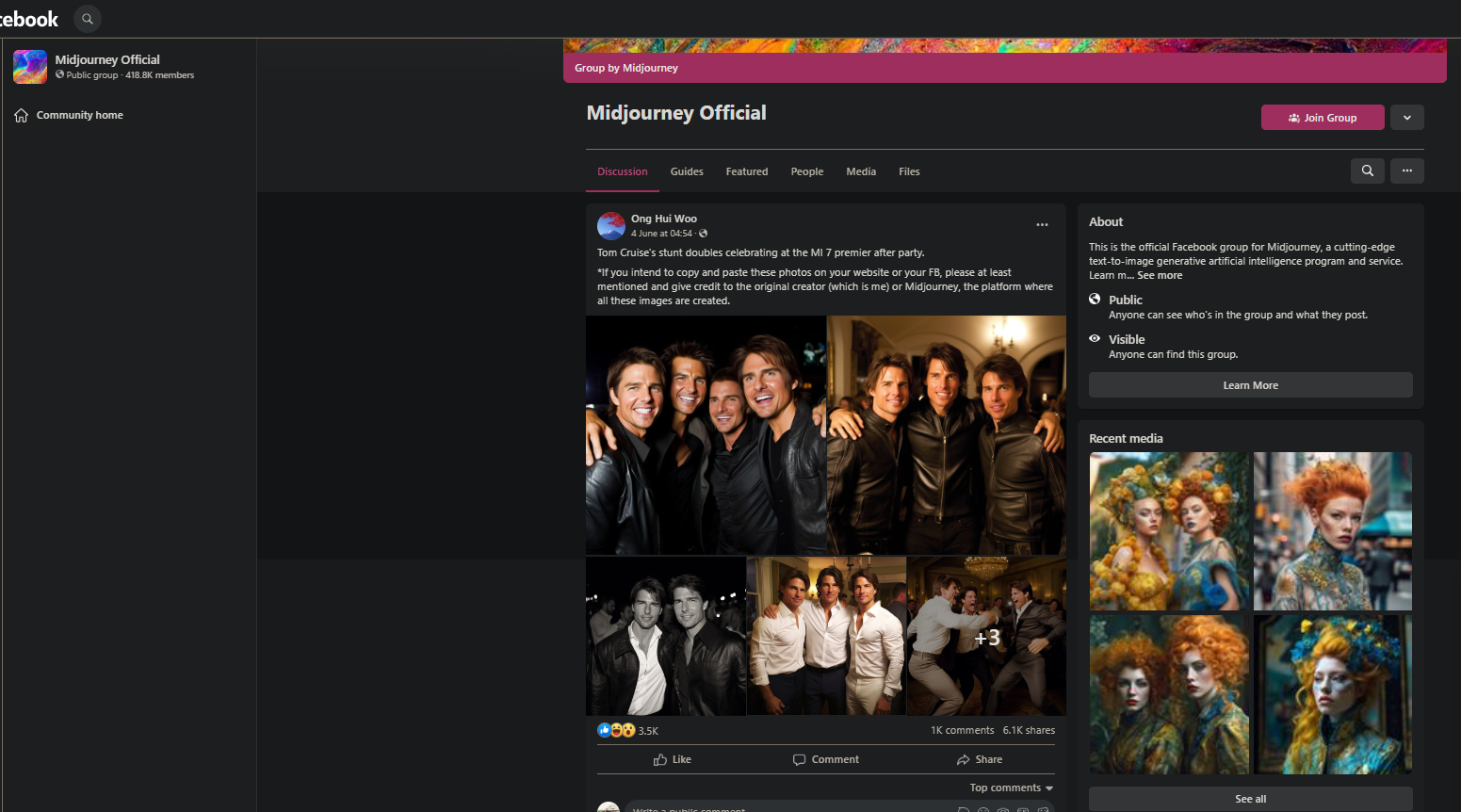This is a detailed screenshot of a Facebook page for the group "Mid-Journey Official." In the upper corners of the screenshot, the term "EBOOK" is visible alongside the group's profile picture. Underneath this image, though the print is too small to read clearly, it likely indicates that the group is public, lists the number of members or followers, and denotes it as the community's home.

The main section of the page begins with a banner in purple stating "Group by Mid-Journey." Below this, there is a "Join Group" button accompanied by a downward arrow, and tabs for navigating through the page: "Mid-Journey Official," "Discussions," "Guides," "Featured People," "Media," and "Files." 

The focal post on the page, written in large text is "ONGHUWOO," and it details an event where Tom Cruise's stunt doubles are celebrating at the M7 premiere allure party. Although the print below this is quite small, the post emphasizes the importance of crediting the original creator if the photos are used elsewhere, specifying that credit should go to either the individual author or Mid-Journey, the platform used to create the images. 

The post is accompanied by several photos depicting Tom Cruise and multiple men who resemble him, presumably his stunt doubles. To the right side of the page, there is an "About" section and some additional photos shared by Mid-Journey.